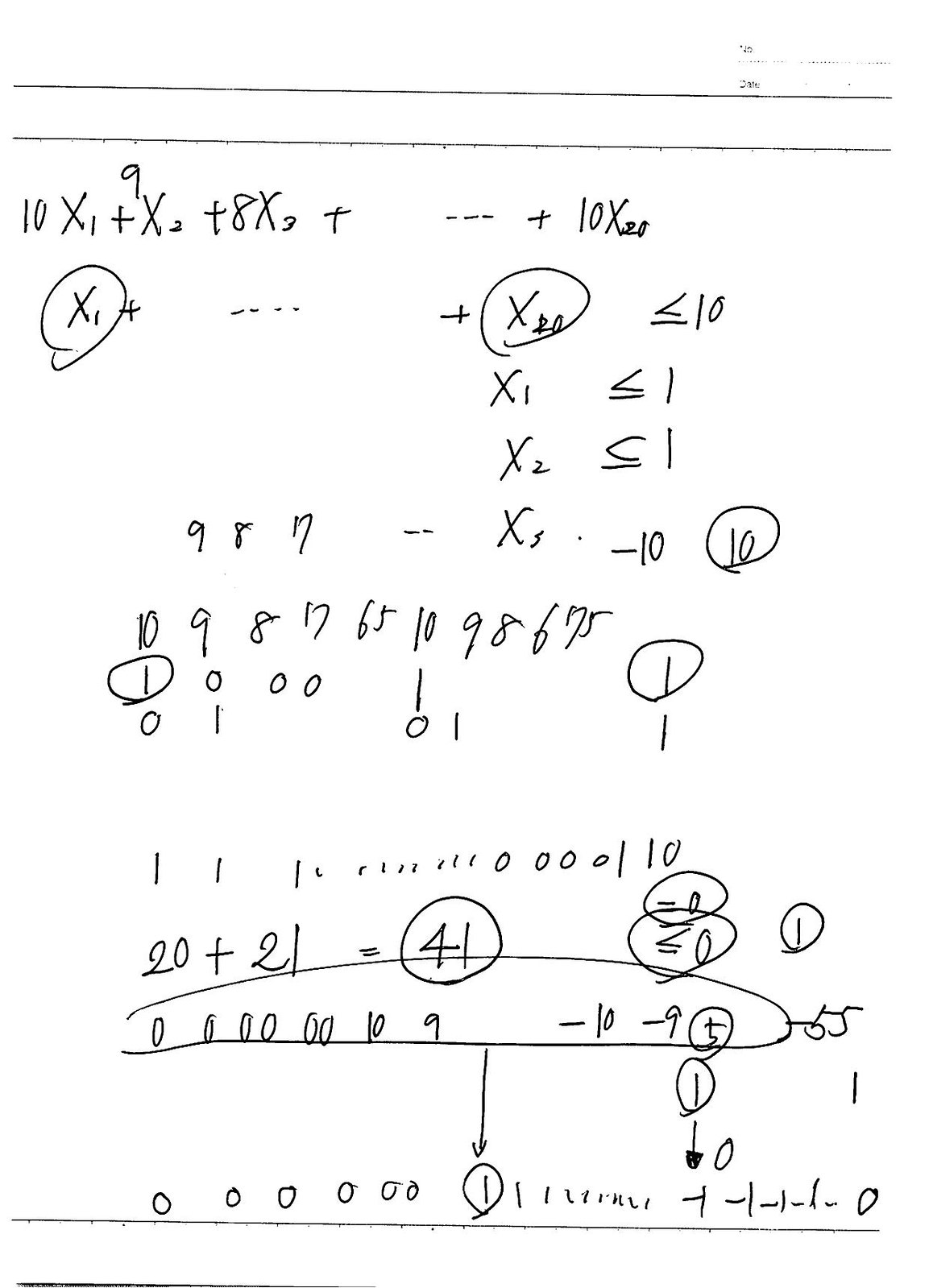The image depicts a sheet of white paper filled with various mathematical equations written in black ink. At the top of the paper, two black lines run horizontally across the width. Near the bottom, another thick black line extends across, but a second black line below it stops halfway from the left edge of the sheet. 

The first equation at the top of the page reads: 
\[10x_1 + 9x_2 + 8x_3\]

Continuing below, there are additional algebraic expressions that conclude with less than or equal to signs, such as:
\[ \text{Some equations} \leq 10 \]

Further down the page, individual constraints are provided:
\[ x_1 \leq 1 \]
\[ x_2 \leq 1 \]

Additionally, another expression appears:
\[ 987...\cdots x_5 - 10 \]

The number 10 is circled prominently near these equations. Scattered below that are more quantities and algebraic notations with no discernible order or systematic structure, giving the impression of random equations jotted across the sheet.